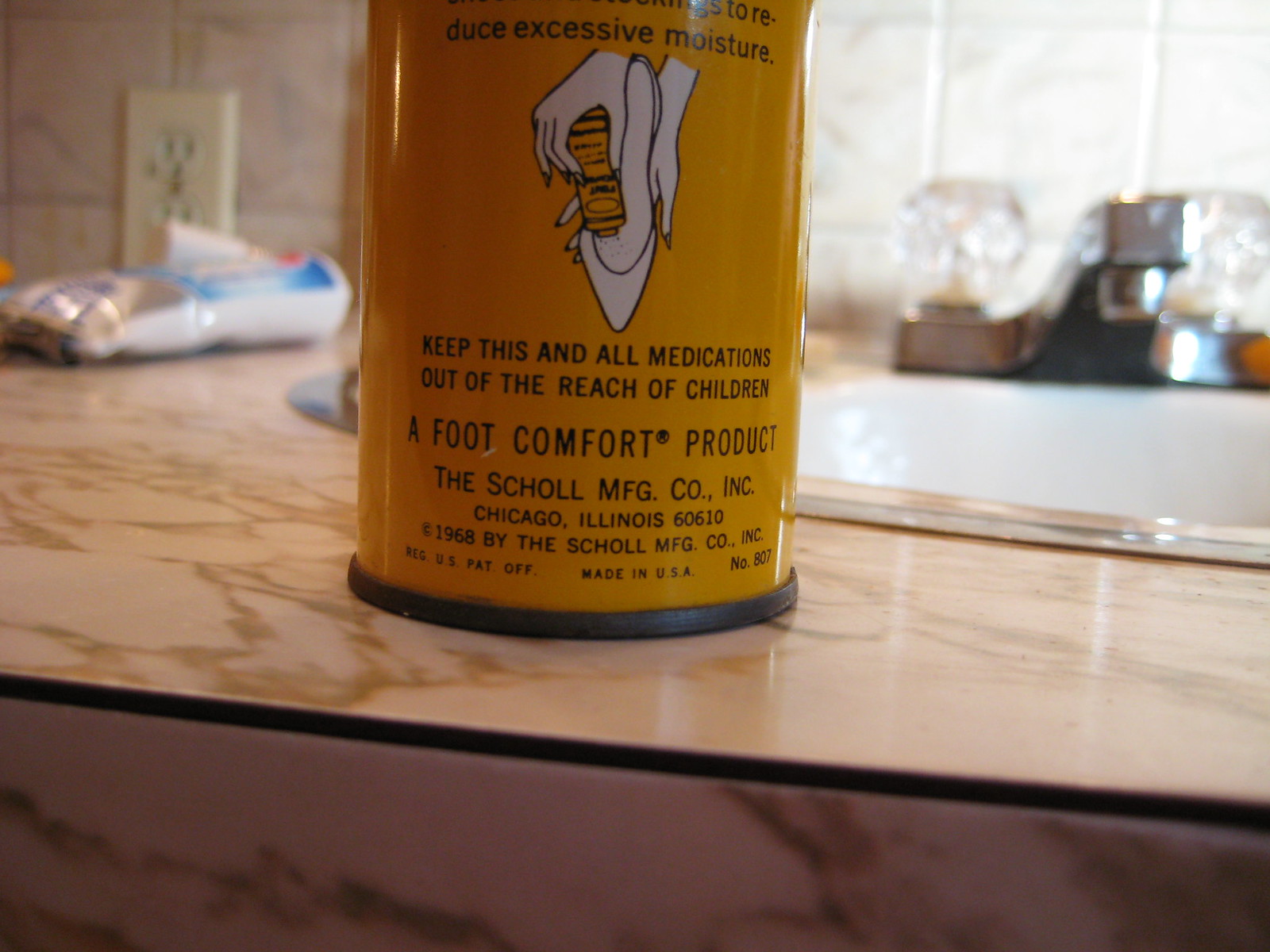In the image, there's a bathroom sink area as the background. The sink itself is white, complemented by a white backsplash. Above the backsplash is a double power outlet with a white cover. To the side, there's a white toothpaste tube featuring blue and red accents. The countertop has a mottled appearance, blending shades of gray and brown. Centrally positioned in the scene is a pair of hands holding a yellowish-brown can. The can's label reads, "Keep this and all medications out of the reach of children." Additionally, it mentions "A foot comfort product" from The Shoal Manufacturing Company, Incorporated. The sink is equipped with a silver faucet and clear handles.